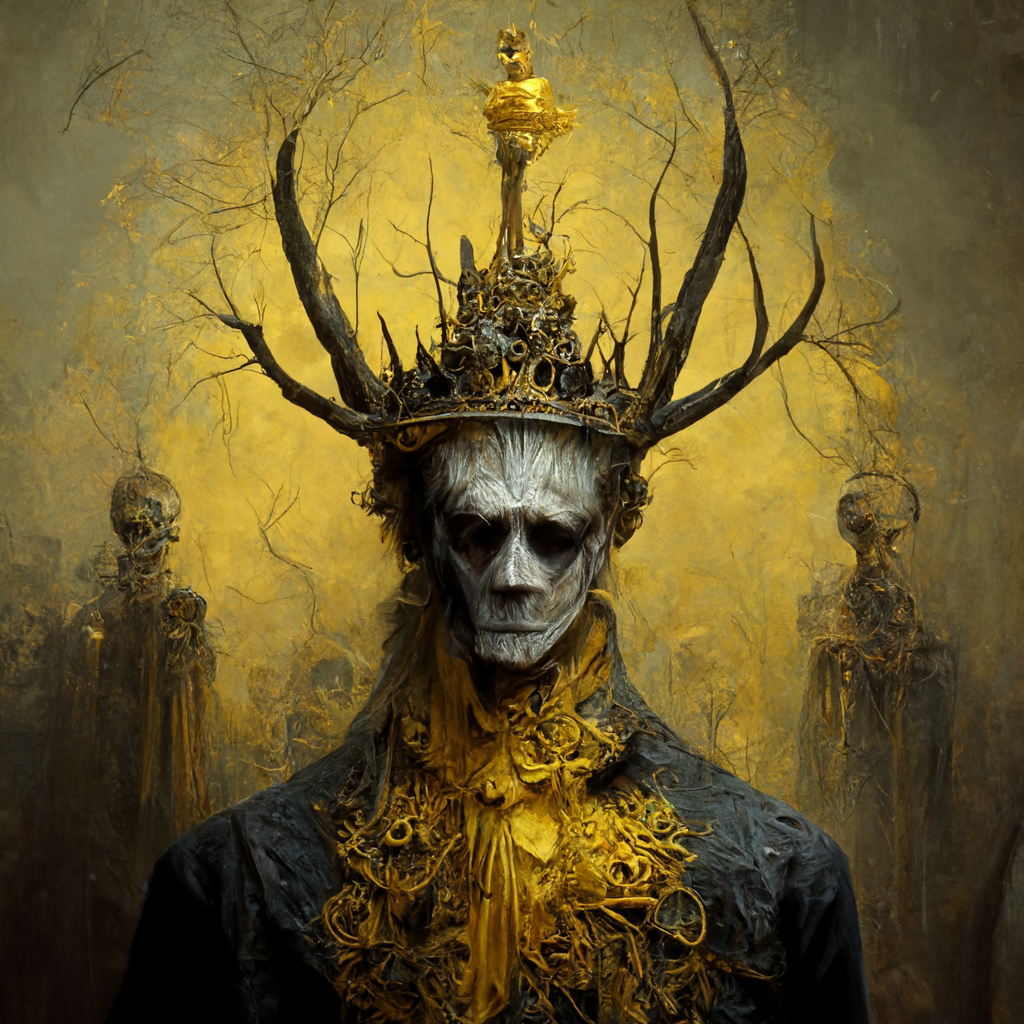The painting features a haunting, horror-movie-like image dominated by a central figure that evokes a decayed, deer-like humanoid. This figure, with an unsettling, gray, and partially decayed face covered in splotches of brown, stares out into the void with hollow black eyes that resemble empty chasms. The skin of the figure appears intact yet eerily lifeless. Atop the figure’s head sits a elaborate crown adorned with antlers and an intricate collection of silver and gold pieces that stack up to a pinnacle, culminating in a long golden piece affixed with various gold nuggets. 

The central figure is clad in an intricately detailed dark blue jacket embellished with gold embroidery along the neckline and front. The sartorial details extend to a large, intricately carved or woven yellow scarf flowing down the chest, adding to the figure's ornate appearance.

Flanking the main character are somewhat indistinguishable, similarly eerie figures with shadowy, indiscernible faces. The background of the painting is in hues of gold and orange, permeated by leafless tree branches that add to the chilling atmosphere. The top corners of the painting fade into darker, olive or gray tones, contributing to the muted, somber color palette. In the background, skeletal, statue-like figures in gold and gray stand like silent sentinels, enhancing the painting's eerie, unsettling vibe.